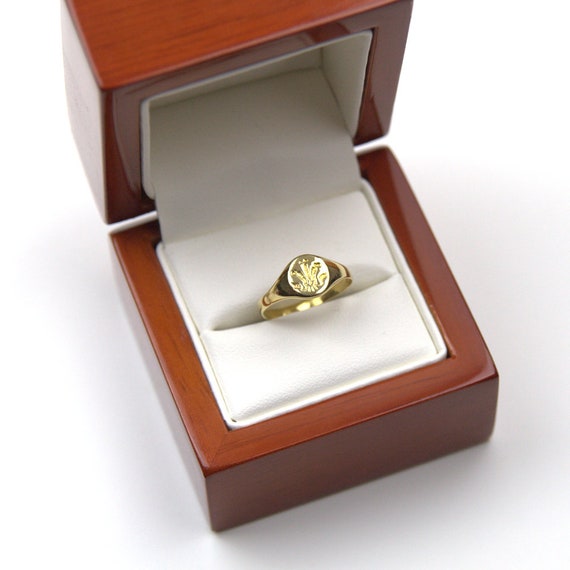This close-up photograph features a gleaming gold ring nestled in an open ring box. The box is made of rich mahogany wood, characterized by its cherry hue and darker grain patterns. The box sits on a solid white surface, creating a stark contrast that highlights its details. Inside, a soft white velvet cushion securely holds the ring. The ring itself, which appears to be a man's pinky ring, boasts a bright gold finish that reflects light brilliantly. The ring's flat top is adorned with an intricate crest or crown emblem, meticulously etched into the gold. The square image has no borders or text, directing full attention to the pristine, new ring and its elegant packaging.